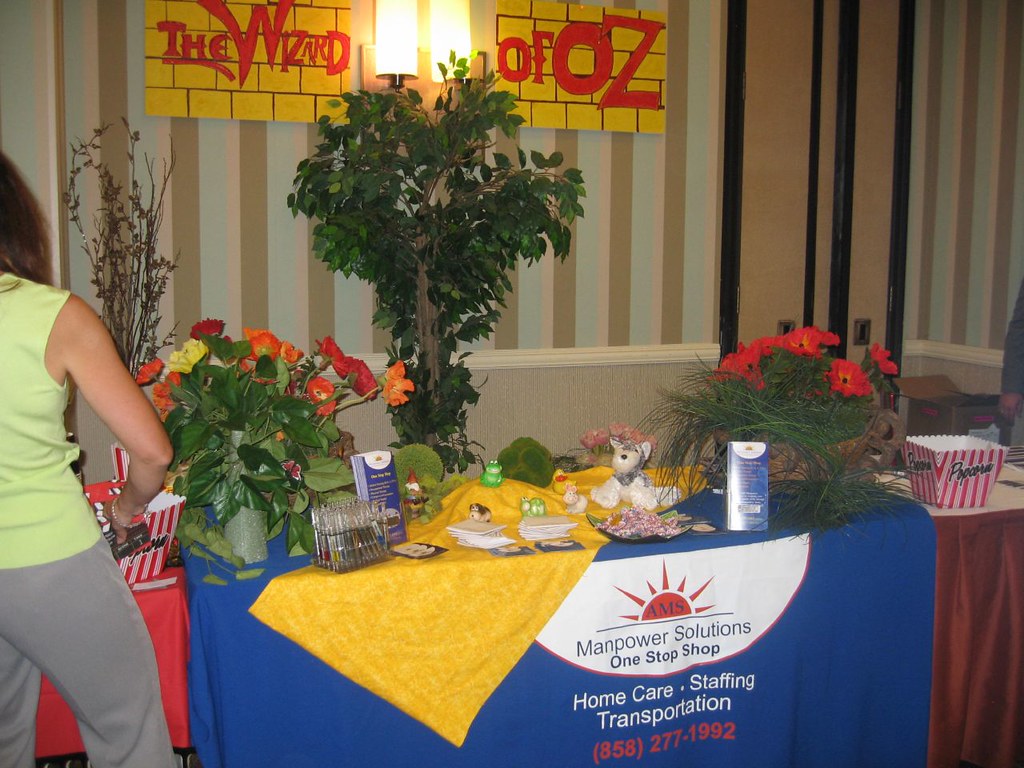The image depicts a lively event setting with various details prominently featured. In the foreground, there's a table draped with a blue cloth, overlaid by a yellow cloth, bearing a prominent banner that reads "Manpower Solutions One Stop Shop" with a logo featuring a red sun over a white half circle. Beneath the logo, it lists services in white text: "Home Care, Staffing, Transportation," accompanied by a phone number in red: "858-277-1992." The table is adorned with bouquets of flowers, stuffed animals (including a dog, pig, and frog), a collection of pens, pamphlets, and what appears to be plastic silverware.

To the left of the table is a woman in a yellow tank top and gray pants, with brown hair, and only the back of her right arm visible. She appears to be engaged with a red and white striped popcorn container, either picking it up or attending to its contents. Behind her stands a ficus tree, adding a touch of greenery to the scene.

In the background, the wall features brown and white vertical stripes and is decorated with signs resembling yellow bricks, evoking the imagery of the Yellow Brick Road from "The Wizard of Oz." The signs are split with "The Wizard" written on the left and "Of Oz" on the right, in bold red letters. The setting seems to blend business promotion with a casual, festive atmosphere, possibly related to a catering or community event.